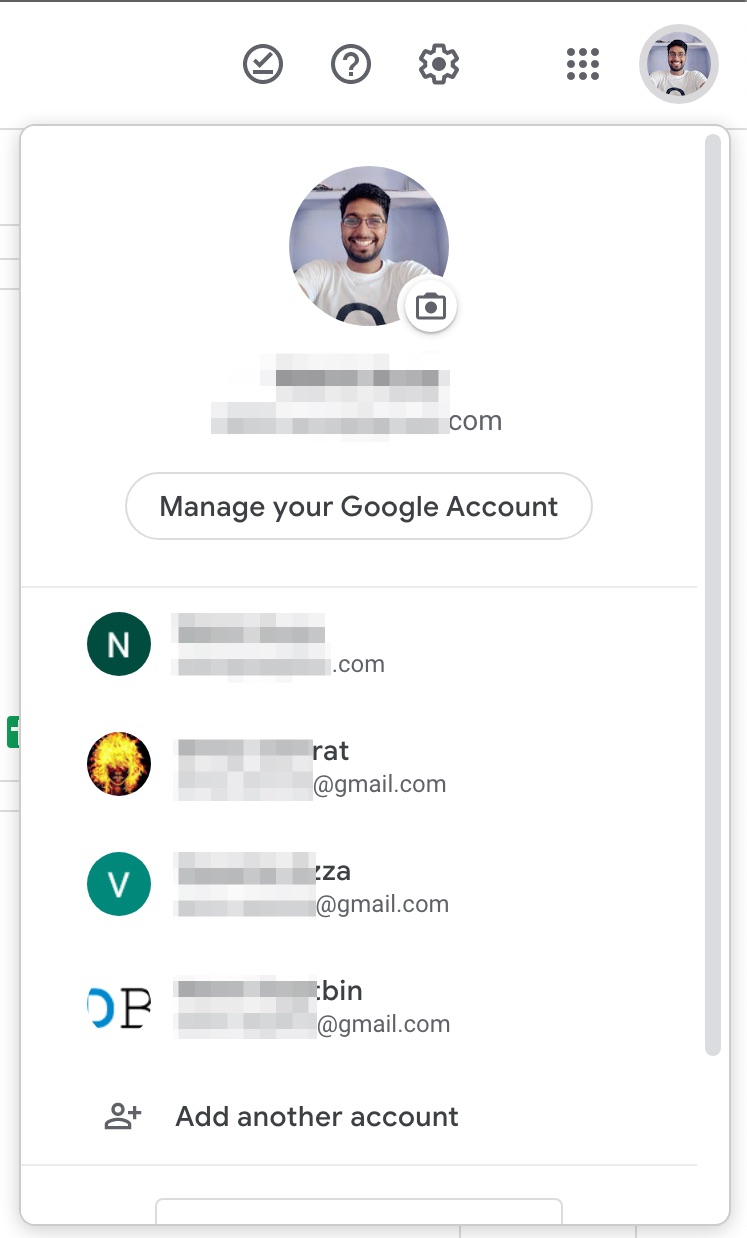This screenshot showcases a mobile application interface with a predominantly white background accented by thin black lines at the top. Central to the image, a collection of icons is displayed, including a check mark, question mark, settings gear, a nine-dot menu symbol, and a small circular profile picture of a man. The profile picture is prominently zoomed in the overlay at the center of the screen, featuring an ethnic man with short black hair and a neatly trimmed beard and mustache. He is smiling and wearing a white shirt. Behind him, a blue circular background can be seen, though it is somewhat obscured.

In the lower right corner of this zoomed-in profile picture, there is a small camera icon next to blurred out text reading "something.com". Below this overlay, a button labeled "Manage your Google Account" is visible.

Further down the screen, there is a list of linked accounts represented by various icons: 
- A green circle featuring a white 'N'
- A black circle with a bright flame inside
- A teal circle displaying a white 'V'
- A white background circle containing a blue 'O' and a black 'B'

All associated usernames or email addresses are blurred, and at the bottom of the list, the option to "Add another account" is present.